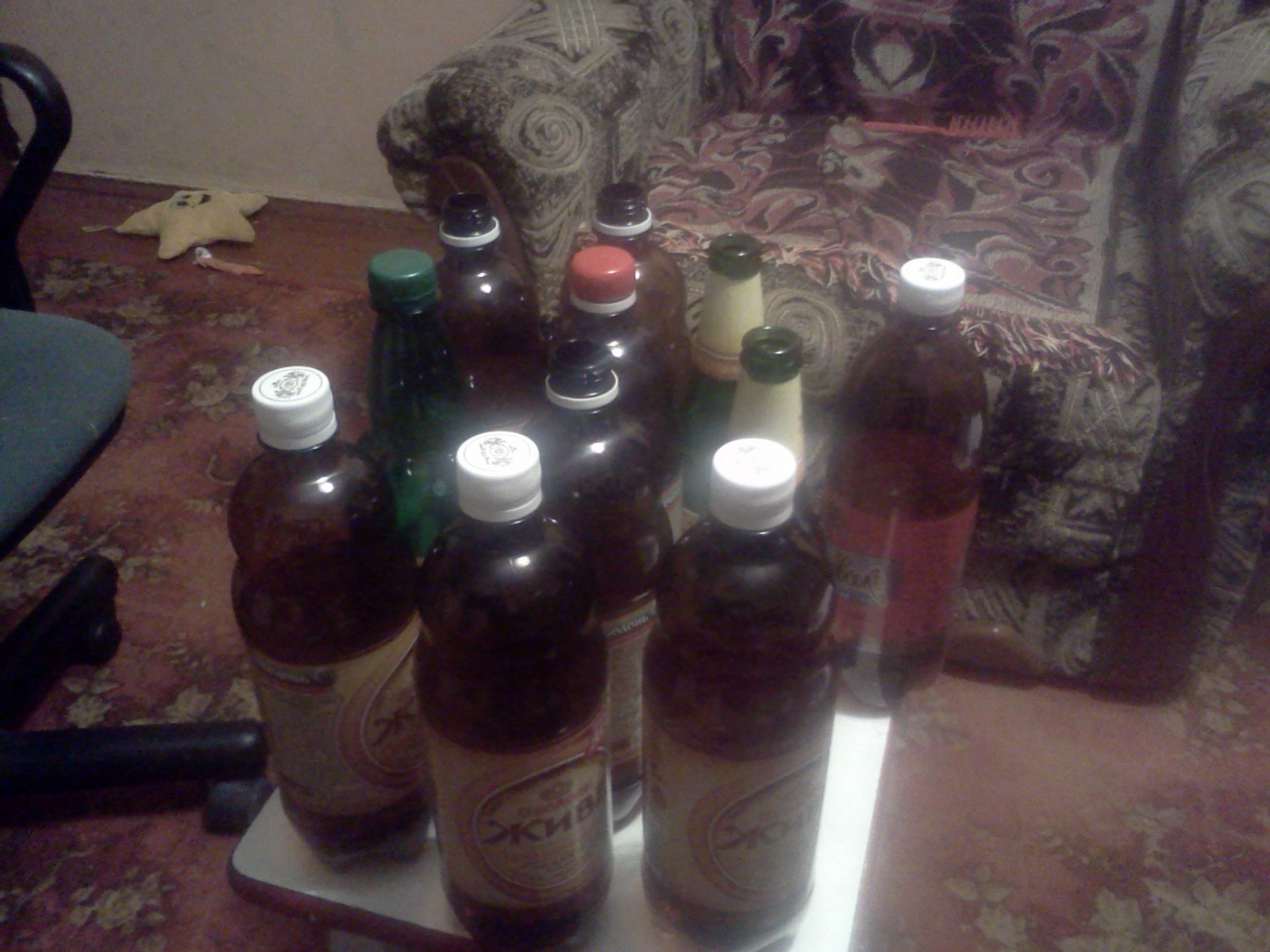The image is a grainy, color snapshot of a dated living room with a worn-out maroon carpet featuring beige floral patterns. At the center of the room, there is a small, white, laminated table cluttered with a mix of plastic and glass bottles, some opened and others still sealed, including one with a white security ring and a mismatched reddish cap. To the right, a fraying, patterned armchair with a blanket draped over it adds to the room's outdated aesthetic. On the left, a blue office chair with black legs and armrests partially enters the frame. The background reveals a hardwood floor meeting the edge of the carpet, a white wall that appears dirty, and a stuffed star toy lying on the floor. The overall scene evokes a sense of neglect and nostalgia, hinting at a space that has seen better days.